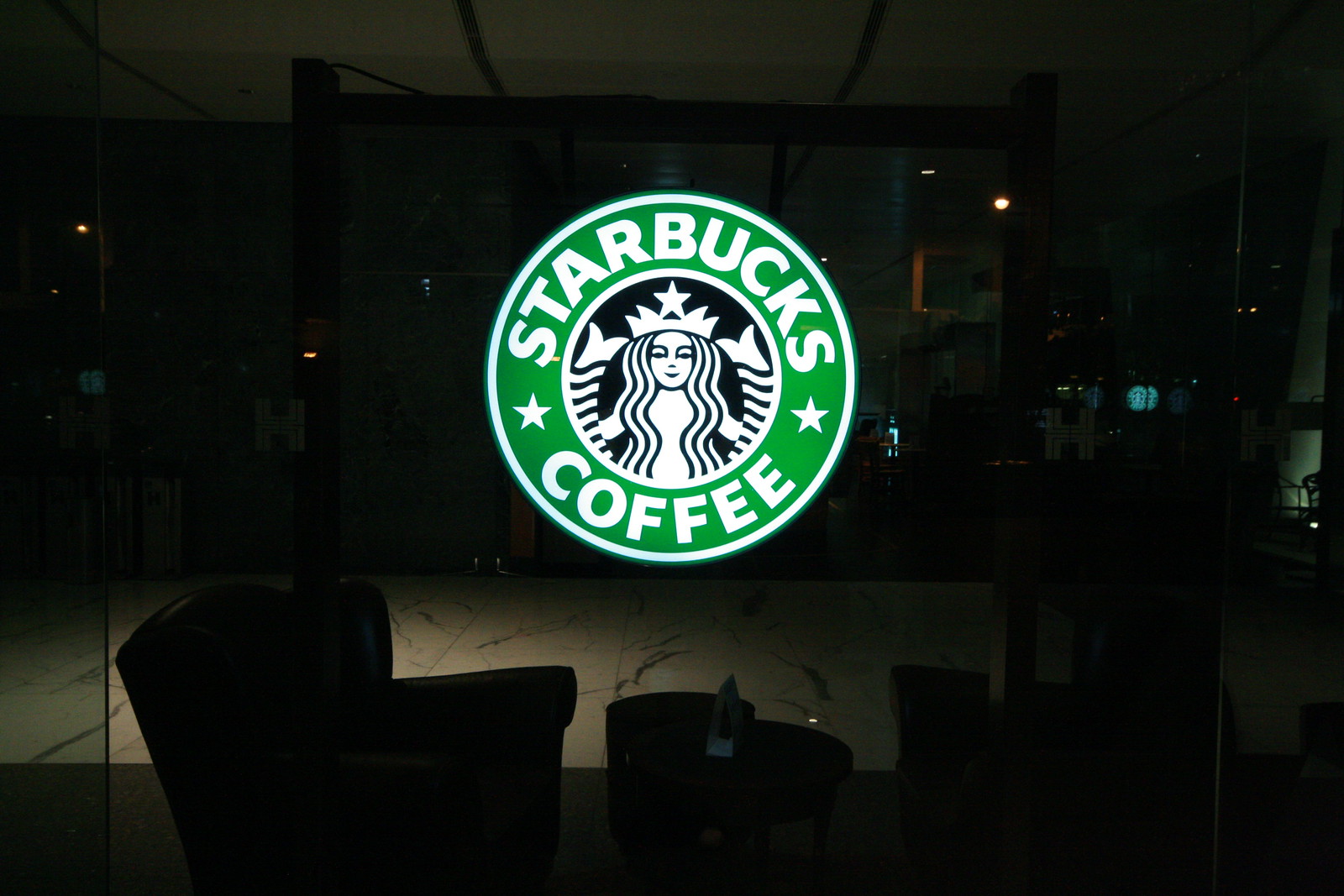The image depicts the inside of a dark, likely closed building with two discernible levels. The focal point of the photo is a large, illuminated Starbucks logo positioned against what appears to be a large glass wall. This iconic logo, predominantly green, white, and black, features a mermaid with a crown and long wavy hair in the middle. Encircling the mermaid is a green ring with "Starbucks" in white capital letters on the upper half, and "Coffee" on the lower half, accompanied by a star on each side. The background is dimly lit, revealing the vague outlines of a white marble floor, chairs, and a coffee table on the lower level. The upper level seems to resemble a studio, but details are hard to discern due to the darkness. Through the glass, the silhouettes of buildings are faintly visible, adding to the nocturnal ambiance.